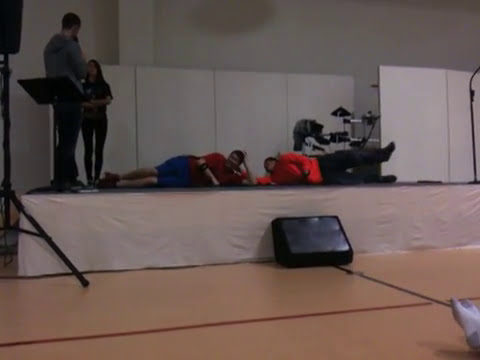This photograph captures an indoor scene with several individuals on and around a small, rudimentary stage that has white borders. The stage itself appears to be set up with various audio equipment, possibly including a large speaker and a tripod stand. There is also a black metal stand for holding notes. On the stage, a girl dressed in all black and a tall man wearing a gray hoodie with jeans stand on the left side; they seem to be possibly conversing. In the center of the stage, two boys are lying down with their heads close together but oriented in opposite directions. One boy wears a red shirt with blue shorts, while the other boy wears a red shirt with black pants. Behind them, toward the back of the stage, there appears to be a drum set. The left side of the stage also features a black suitcase or briefcase placed on the floor. The room itself has light brown flooring akin to a gymnasium, and the walls are mainly white with some gray. One intriguing detail is a person visible in the scene wearing just a pair of socks.